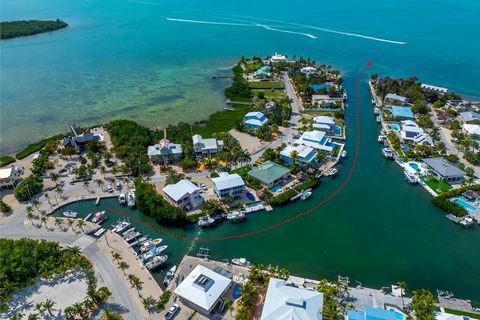The aerial image showcases a densely populated area characterized by a network of narrow waterways and small islands. The top portion of the photograph features a body of water with a greenish tint, possibly due to algae, and is traversed by boats or jet skis, evident from the white streaks on the surface. In the upper left corner, there is a small island, a patch of green land amidst the water.

The central and bottom sections of the image reveal a developed area with a mix of streets, houses, and abundant greenery. The streets, lined with palm trees, curve and intertwine around the waterways. Houses with varied colorful rooftops, some white and green, border these canals, and many have boats docked along the water's edge. In the lower left corner, a road runs parallel to the water, with boats parked beside it.

Scattered throughout the image, particularly in the lower portion, are clusters of buildings, possibly around a marina. The buildings are surrounded by a mix of trees and shrubs, adding to the lush, green appearance of the area. The landscape provides a striking contrast between the greenery of the land and the expansive, open water at the top of the picture.